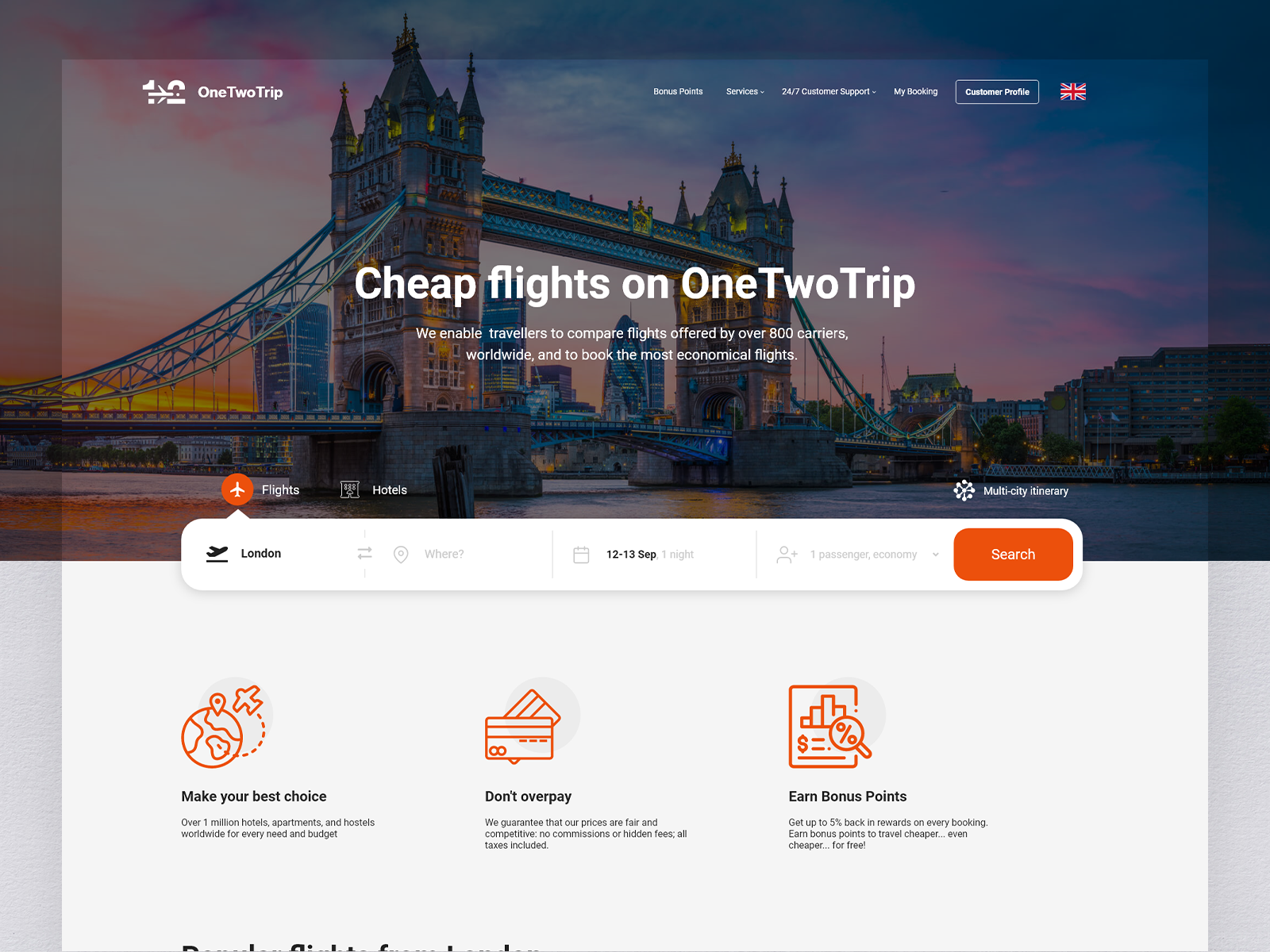The webpage layout for "1-2-Trip" is displayed with a clear, user-friendly design. 

**Header Section:**

- **Top Left Corner:** The site name, "1-2-Trip," is presented prominently in white text. The logo creatively incorporates an airplane icon placed between the numbers 1 and 2.
- **Top Right Corner:** A series of navigational tabs are also in white, listing options like "Bonus Points," "Services," "24x7 Customer Support," "My Booking," and "Customer Profile." Adjacent to these tabs is a UK flag in blue, red, and white, indicating language or region selection.

**Main Body:**

- **Hero Text:** Centrally displayed in white text is a promotional headline: "Cheap Flights on 1-2-Trip. We enable travelers to compare flights offered by over 800 carriers worldwide and book the most economical flight."
  
- **Search Bar:** Just below the promotional text, a comprehensive search bar allows users to input their departure and arrival locations, select dates and the number of nights, specify the number of passengers, and utilize a prominent orange "Search" button on the right side.

- **Left Panel:** Underneath the search bar, a section encourages users to "Make Your Best Choice" by browsing through accommodations with 1 million hotels, apartments, and hostels worldwide to suit every need and budget.

- **Central Panel:** A message ensures users that they "Don't Overpay" with a guarantee of fair and competitive prices, no hidden fees, and all taxes included.

- **Right Panel:** There's a note on earning bonuses, highlighting the opportunity to get up to a 5% banking reward on every booking, along with bonus points to make future travels even cheaper.

- **Bottom Half:** The background transitions to white, in contrast to the top half of the page.

**Banner Image:**
 
- **Top Half:** A visually appealing banner features a suspension bridge over water, set against a vibrant sky with hues of purple and yellow, embellished with darker shades, enriching the overall aesthetic.

This detailed layout emphasizes ease of use and transparency for travelers seeking budget-friendly flights and accommodations.